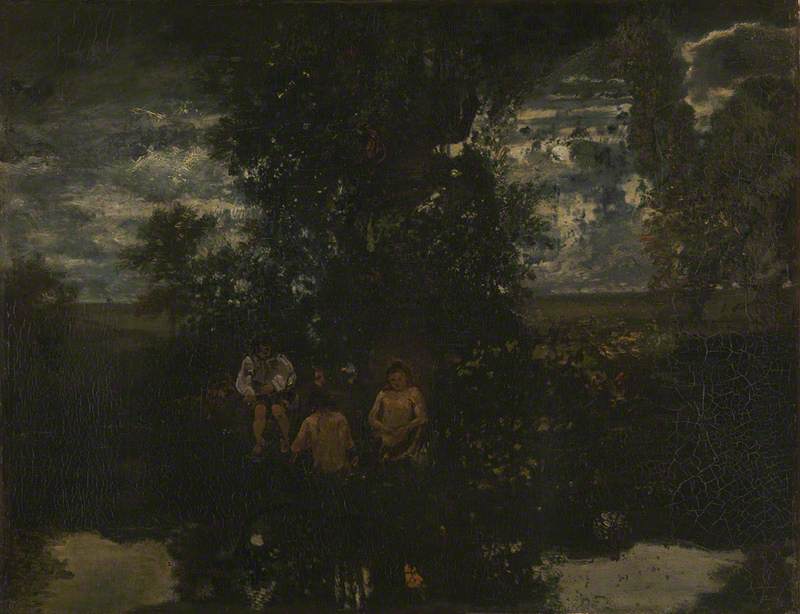The artwork is a hand-drawn painting that captures a serene, yet somewhat eerie night-time scene in a lush, densely vegetated area, reminiscent of a secluded spot deep in the woods. The focal point of the painting is a large, dark-green tree that stands prominently in the center, its branches extending skyward under a cloudy, partly blue sky. Surrounding the tree is a rich array of vegetation, with flowers dotting the landscape in and around the water at the bottom of the image, which also reflects elements from above, creating a mirrored effect.

In front of the central tree are three figures, presumably children, whose presence evokes a sense of innocence juxtaposed with the dark setting. Two of the children appear to be unclothed, their bodies blending with the surrounding dimness. The third child wears light-colored clothing consisting of a long-sleeved shirt and shorts. The arrangement of these children differs slightly between each observer’s perspective, yet all indicate their positions near or within the water, with one potentially sitting on a bank.

Despite the painting's darkness, there is a subtle interplay of light and shadow, particularly around the edges where patches of light escape through gaps in the foliage. The worn and creased texture of the drawing suggests it has been frequently handled, adding to its vintage and mysterious allure. Overall, the scene portrays an enigmatic moment frozen in time, set against a backdrop of natural beauty interwoven with a slightly haunting atmosphere.